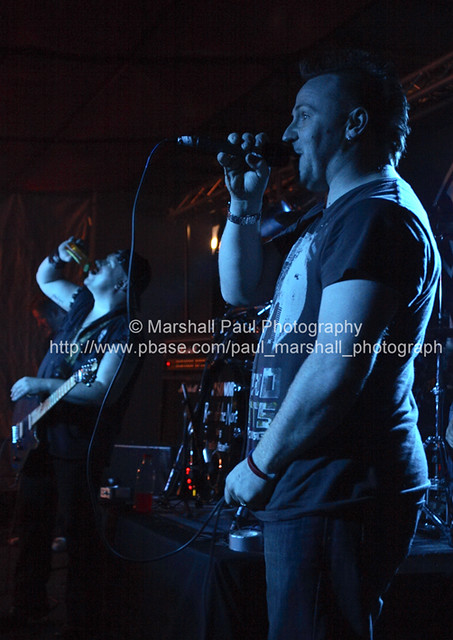The photograph captures a live music performance in a dimly lit venue with a bluish tint, suggesting a club setting. Dominating the right half of the image is a slightly balding, heavy-set man in his 40s, holding a black microphone to his mouth with his right hand while wearing a dark graphic t-shirt and jeans. His short brown hair is visible, and he sports a watch on his right wrist. The man is positioned side-on, facing the audience, adding a dynamic element to the scene. To the left and slightly behind him, another band member appears to be drinking a beer from a bottle, his guitar slung over his shoulders but not being played at the moment. The drinker rests his left hand on the bridge of his guitar, reinforcing the casual, authentic atmosphere of the performance. The backdrop features partial visibility of a drum set, hinting at the presence of a drummer. Across the center of the image, the watermark "Marshall Paul Photography" appears in white font, along with the website "http://www.pbase.com/Paul_Marshall_Photograph," firmly branding the photograph. Red lighting also subtly punctuates the scene, enhancing the overall ambience.